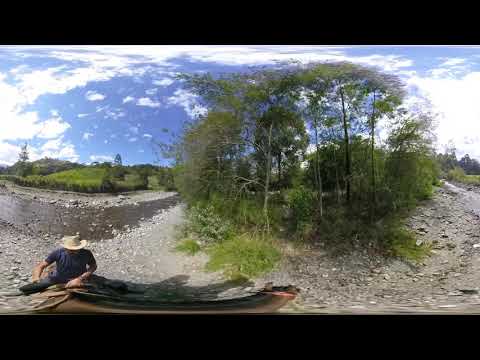The photograph captures a serene outdoor scene during daytime, featuring a man wearing a straw-colored hat and a navy blue long-sleeve shirt. He is seated on the ground near the left bottom corner of the image, close to what looks like a small boat or canoe. Surrounding him is a tranquil setting with shallow, clear stream water flowing through a rocky, slightly muddy area. To the right, a group of thin, bright green trees stands, partially encircling the man. The backdrop is filled with lush greenery, with more trees and plants stretching towards the left, under a rich blue sky sprinkled with a few dispersed white clouds. Sunlight bathes the entire scene, enhancing the peaceful and picturesque quality of the river or stream bank environment.